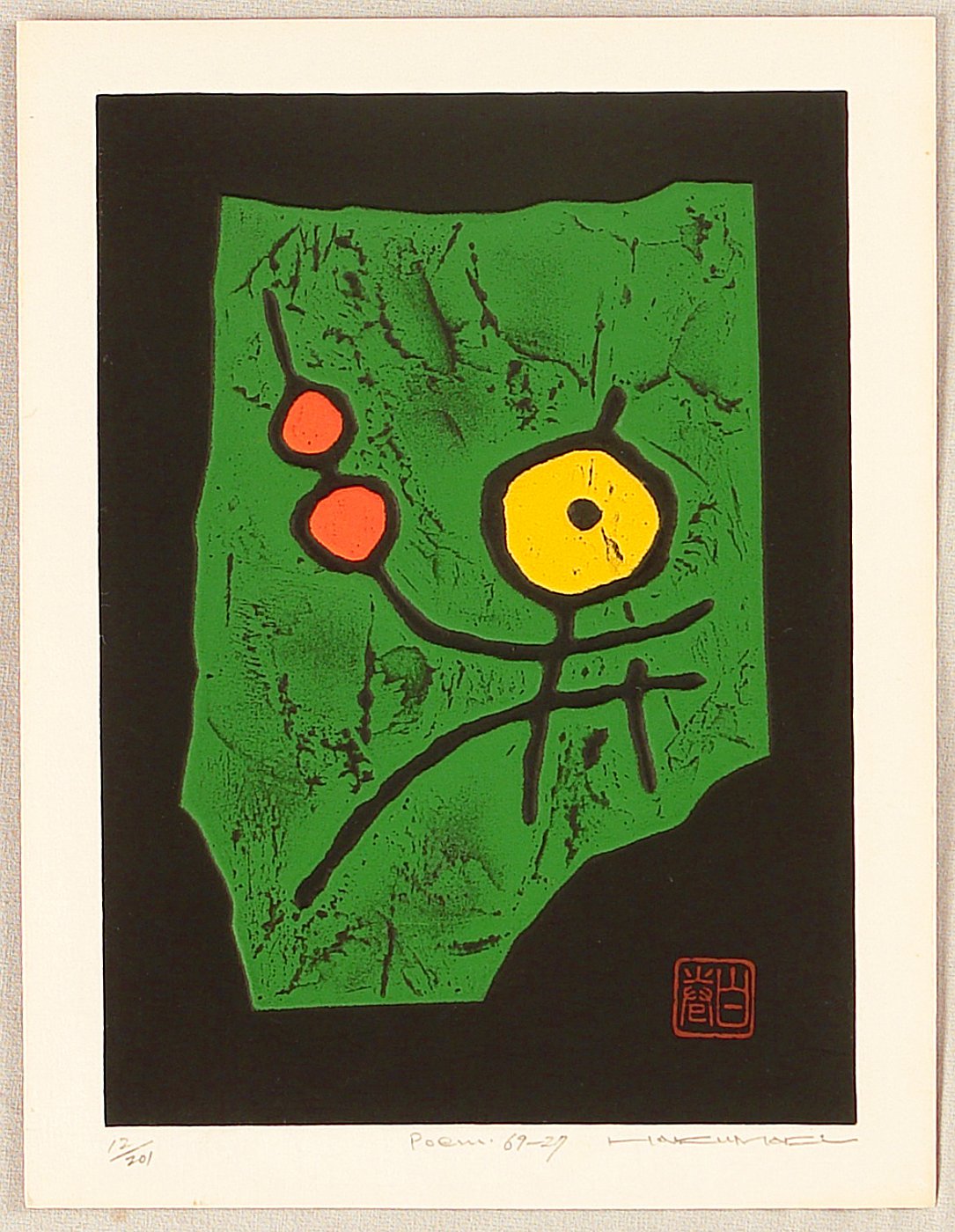The image is a framed drawing with a beige wooden frame. Inside the frame, the outer edge is creamy in color, transitioning to a black background. At the center of the piece, there is an irregularly shaped green area, reminiscent of a Stone Age style, with hints of black. The green area is longer at the top, tapering towards the bottom with cutouts on the lower right and left. In the middle of this green expanse, a stick figure is depicted. The figure's body is formed by black lines, with an oversized, yellow circle for a head, featuring a black dot at its center, suggesting an eye. This stick figure comes across as human-like, or perhaps even a phoenix, with two orange (or red) circular shapes connected by a black line, which the figure holds aloft with its long left arm. The stick figure has a short right arm, a very long left leg, and a much shorter right leg, giving the impression it is sitting or positioned creatively. The simplistic yet captivating style evokes a primitive, almost logo-like quality, underscored by a small signature or logo in the lower right-hand corner of the green area.